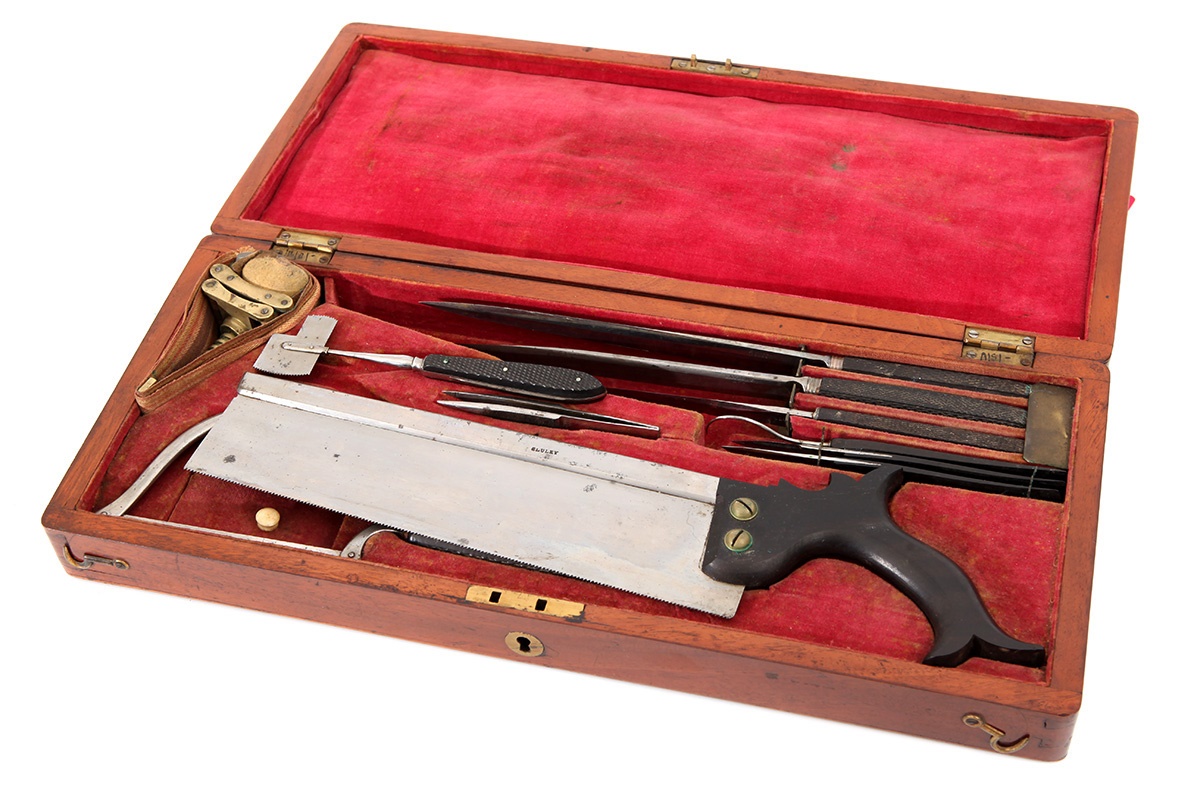This detailed photograph captures a finely crafted antique surgery set housed in an ornate wooden box adorned with gold ornamentations. The box, which is custom-made for its contents, features a keyhole and two metallic yellow latches on the front and is lined with plush red velvet fabric. Inside, a variety of old-time surgical implements are meticulously arranged. Central to the collection is a large surgical saw with the word "CLULI" engraved on the top of its metal blade, which is securely fastened to a dark wooden handle by two prominent golden screws. Alongside the saw, there are additional metallic tools, including a second saw, various knives, cutters, and a pair of silver tweezers. These tools, whose specific uses might be unclear to a layperson, reflect a historical era of medical practice and craftsmanship.